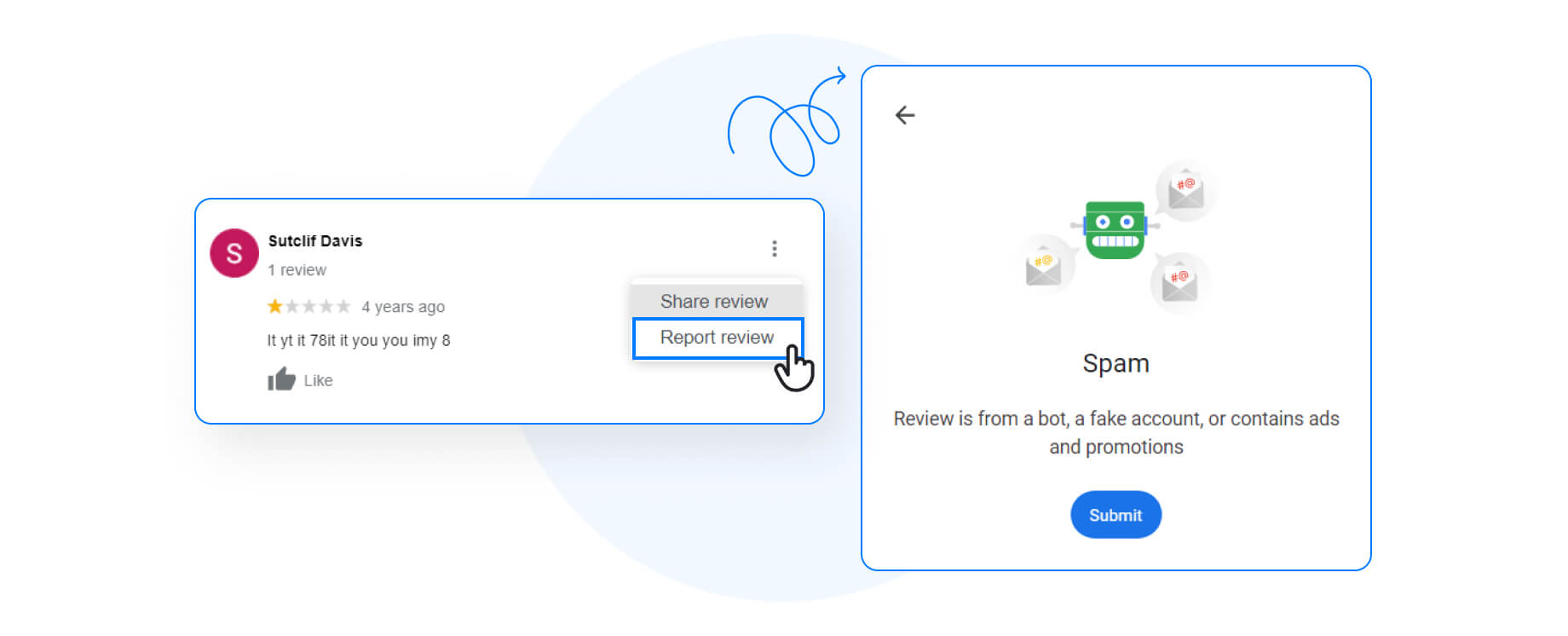The image appears to be a partial screenshot likely taken from a laptop screen. On the left side, there is a box displaying the name "Sutcliffe Davis" accompanied by a purple circle containing the letter "S". Beneath the name, it shows "One Review" along with a one-star rating posted four years ago. Below this, there is text that appears to start with "ItYT," followed by a faded-out like button.

To the right of this review section, there is an option to "Share Review," and just below it, "Report Review," which is highlighted with a blue border around the rectangle.

Towards the middle top of the image, there is a squiggly line ending in an arrow pointing to another box on the right side. This box contains character icons, one resembling a robot and three resembling envelopes. The text beneath them reads "Spam," indicating that the review may be from a bot, a fake account, or contains ads and promotions.

Underneath this description, there is a blue button labeled "Submit."

In the background, a large, faded gray circle is visible, with the remainder of the background being predominantly white.